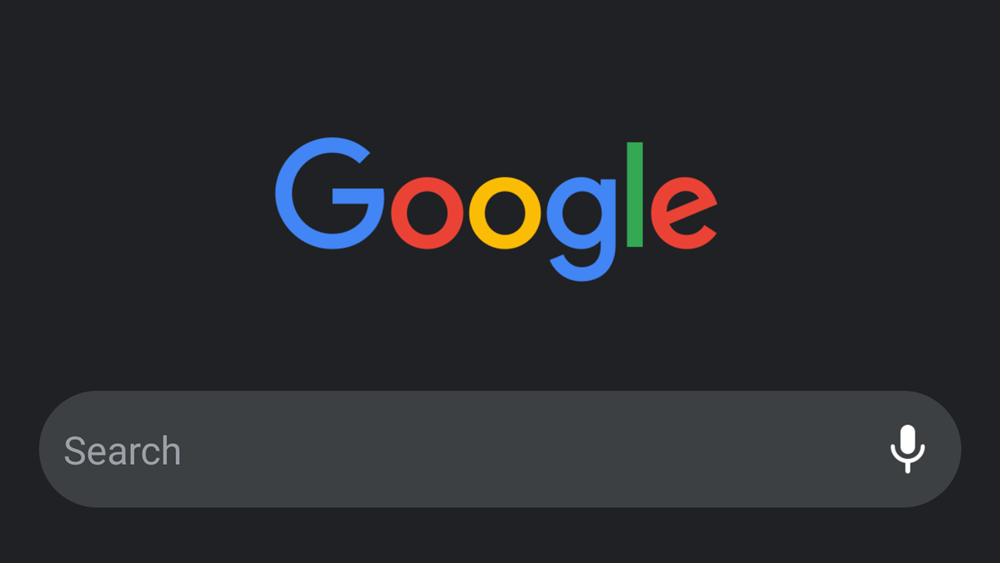The image is a simple and minimalistic screenshot of a portion of the Google homepage, captured in night mode. The entire background is a deep black, highlighting the central colorful Google logo. The logo spells out "Google" with a blue uppercase 'G', a red lowercase 'o', a yellow lowercase 'o', a blue lowercase 'g', a green lowercase 'l', and a red lowercase 'e'. Below the logo, there is a horizontally oriented cylindrical search bar. On the left side of the search bar, the word "Search" is displayed in gray with a capital 'S'. On the far right of the search bar, there is a white microphone icon, indicating the option for voice search. The rest of the page is empty, devoid of any additional elements such as settings, images, or login options, emphasizing a clean and bare interface. This focused capture isolates the core components of the Google search experience against a stark, black background.